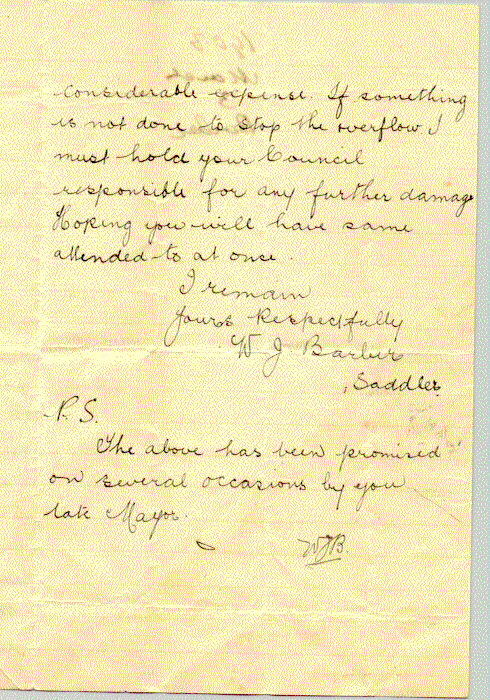The image depicts an old, yellowed piece of paper, showing signs of having been squashed and then straightened, with noticeable dents and creases. The paper features black cursive handwriting, making it difficult to decipher. Despite the overall unreadability, it is clear that the letter is personal and written in English. Key legible phrases include a statement towards the end reading, "I remain yours respectfully," followed by the initials or name "W.J. Barbara Sadler." Additionally, there is a postscript at the bottom that mentions, "P.S. Bob has been performed on several occasions by you," and a signature that looks like "Lally Mayer." The distressed and crinkled state of the note, coupled with its aged appearance, suggests it has been handled multiple times, adding to its historical feel.